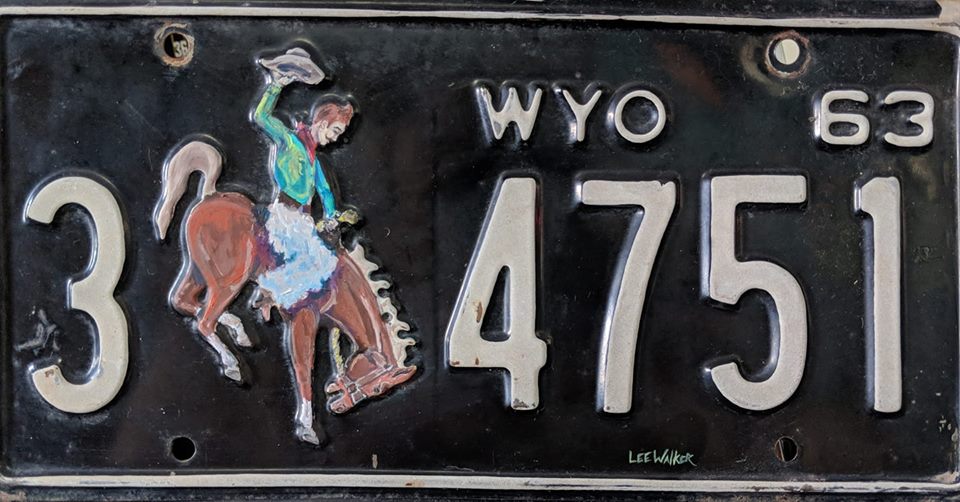This close-up photograph captures an old Wyoming license plate from 1963, filling the entire frame. The plate features a black background with white stamped lettering and a white border, showing signs of age with rusty holes where screws would be placed. At the top, the plate reads "WYO 63" in small white letters. The main focus is the large license number "3 4", followed by a detailed image of a cowboy riding a bucking bronco. The brown horse is depicted with its legs kicking up and its head down. The cowboy, with brown hair, wears a blue-green shirt, blue pants, a red handkerchief, and a beige hat that he holds high in the air. The sequence continues with the numbers "7 5 1". At the bottom in light green, the name "Lee Walker" is inscribed in very small print.